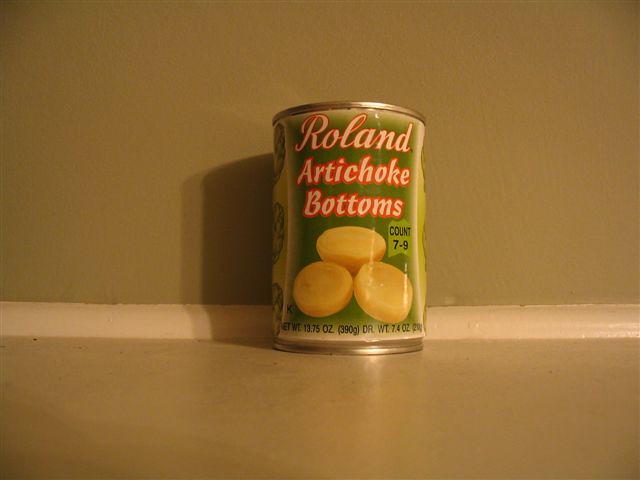In this rectangular image, a can of Roland Artichoke Bottoms is prominently featured. The can, which appears to be made of either aluminum or steel, contains 7 to 9 artichoke bottoms with a net weight of 13.75 ounces when drained. The label is a rich green color, adorned with the words "Roland Artichoke Bottoms" in elegant white script that is outlined in red. A photograph of three artichoke bottoms is displayed on the front of the can, showcasing the product inside. The can is positioned centrally on what seems to be a brown floor, though it could potentially be a shelf, as the surface matches the brown color of the back wall or container holder. Along this wall runs a thin strip of white molding, adding a simple yet clean detail to the background. The can's placement ensures it is the focal point of the image, drawing attention to the brand and product being showcased.